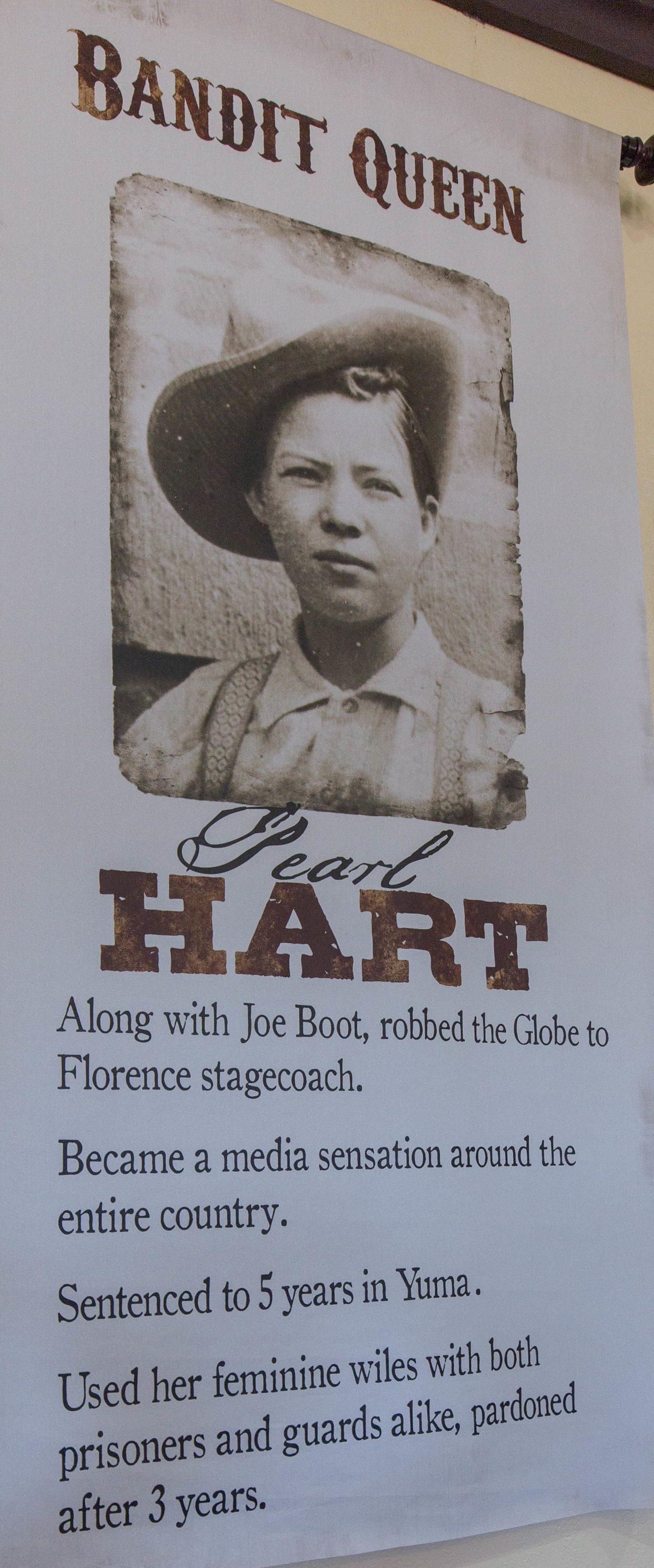The image depicts a vintage-style poster or banner, likely mounted on a wall, which prominently features the title "Bandit Queen" in bold capital letters at the top. Below this title, there is an old black-and-white photograph of a woman donning a hat typical of the stagecoach era, identified as Pearl Hart. The name "Pearl" is written in an elegant cursive font, while "Hart" is rendered in big, bold, red capital letters. The poster provides a brief historical account, stating that Pearl Hart, along with Joe Boot, famously robbed the Globe to Florence Stagecoach, a crime that captivated media attention nationwide. The text further details Hart's subsequent five-year sentence in Yuma, noting that she used her feminine charms effectively with both prisoners and guards, leading to her release after three years. The broader layout suggests the poster might be contained within a frame or held up scroll-style, with visible parts of a white background, hints of a black hanging mechanism on the top right edge, and possibly elements of a wooden structure or off-white wall in the background.